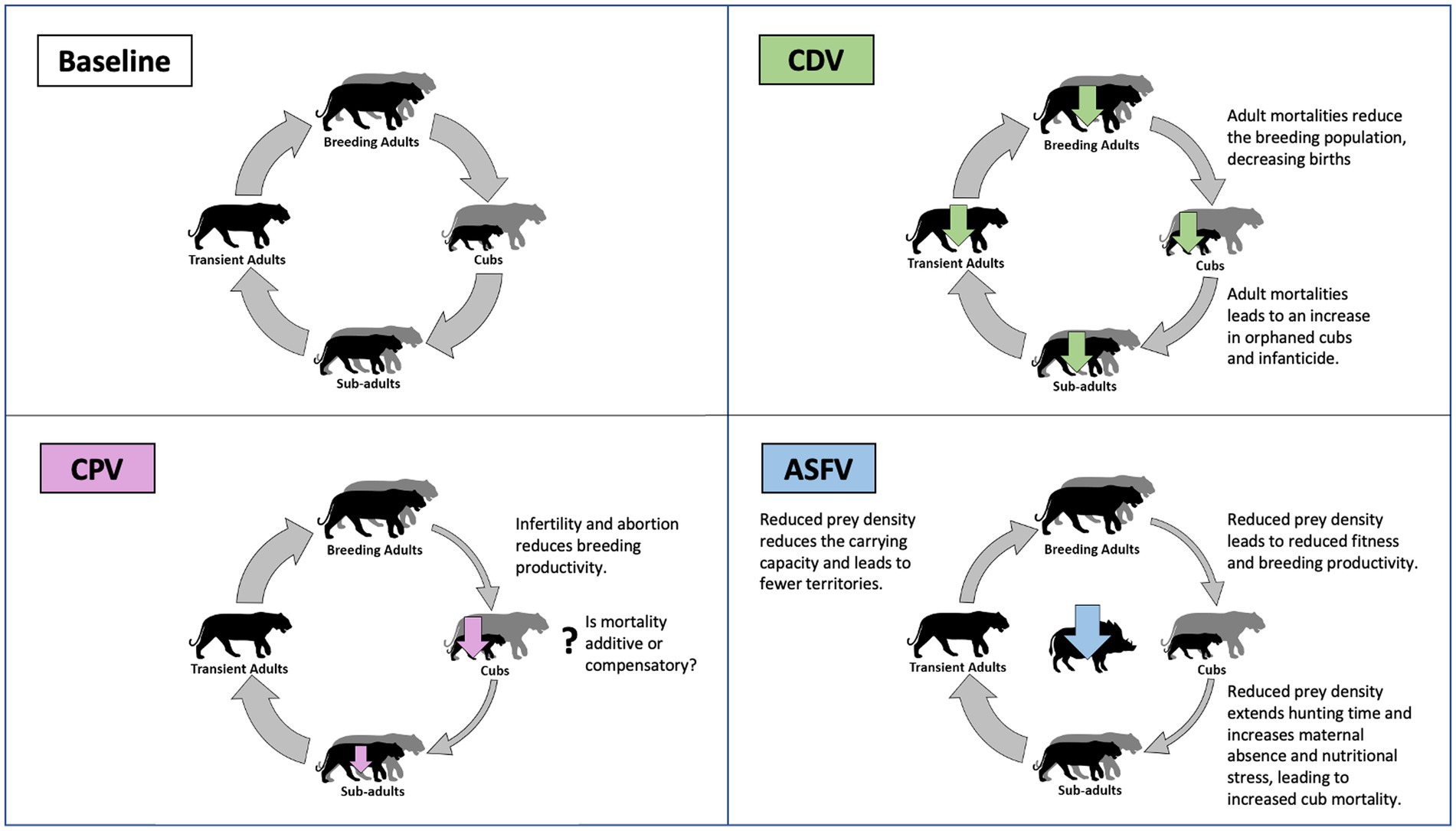This illustration, likely intended for a textbook or educational material on large cats, is organized into a grid of four diagrams, each represented by silhouettes and text in various colors such as green, pink, and blue. The diagrams collectively depict the life cycle and challenges faced by tiger populations:

1. **Top Left (Baseline)**: Shows the standard life cycle of tigers, labeled stages include breeding adults, cubs, sub-adults, and transient adults, illustrating a continuous cycle.
2. **Top Right (CDV)**: Illustrates how adult mortalities affect the population, reducing the number of breeding adults, which in turn decreases birth rates. It points out the subsequent effects such as an increase in orphaned cubs and instances of infanticide.
3. **Bottom Left (CPV)**: Discusses the impact of factors such as infertility and abortion on breeding productivity. It poses a question about whether mortality is additive or compensatory for the tiger population.
4. **Bottom Right (ASFE)**: Focuses on the effects of prey density on tigers' fitness and breeding productivity. Reduced prey density is shown to decrease the carrying capacity, extend hunting times, and increase maternal absence and nutritional stress, leading to higher cub mortality. This diagram features the silhouette of a warthog, indicating it as a prey species.

The entire illustration is in black and white, using silhouettes of tigers and descriptive text to convey scientific data about the species' life processes and survival challenges.